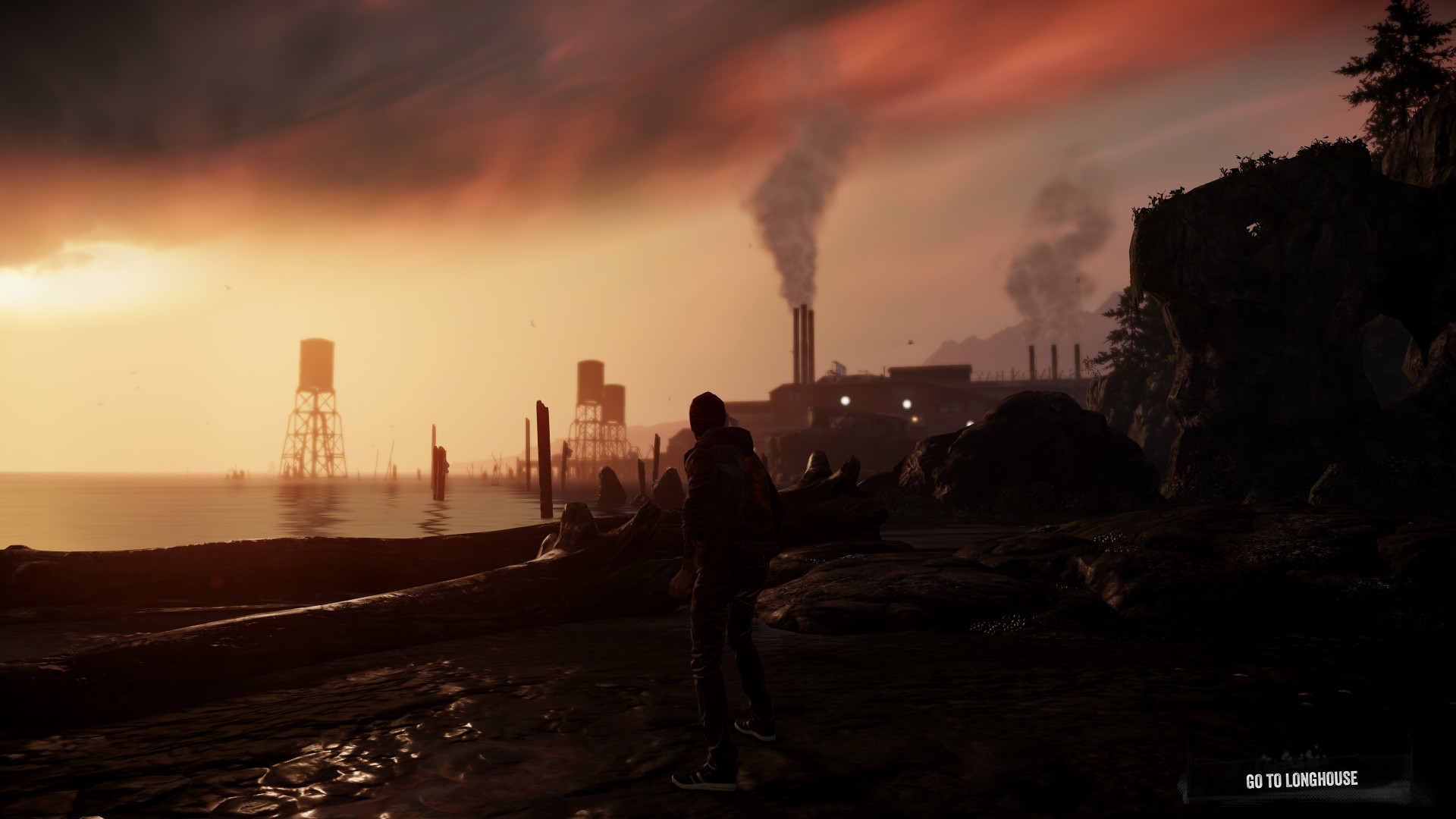This is a dark and moody painting of an industrial waterfront scene, infused with dystopian overtones. In the foreground, several people, including a young boy in sneakers, jeans, and a hoodie, stand or sit on a rocky shore. The water’s edge is marked by posts protruding from the lake or ocean. The people are silhouetted against an eerie, industrial backdrop dominated by factories and oil or water tanks. Smokestacks with billowing plumes of smoke rise prominently, blending into a sky painted with layers of shadows—shades of yellow at the horizon transition to orange, pink, and deep brown as they recede into a darker, more overcast top left corner. The sun struggles to shine through heavy clouds on the right, casting a faint reflection on the water. The air appears thick and polluted, tinged with unsettling hues of orange and brown. Reflective surfaces in the water mirror the towers and add to the overall sense of desolation. In the bottom right-hand corner, the phrase "GO TO LONG HOUSE" is displayed in white capital letters, offering an enigmatic directive amidst the somber scene.